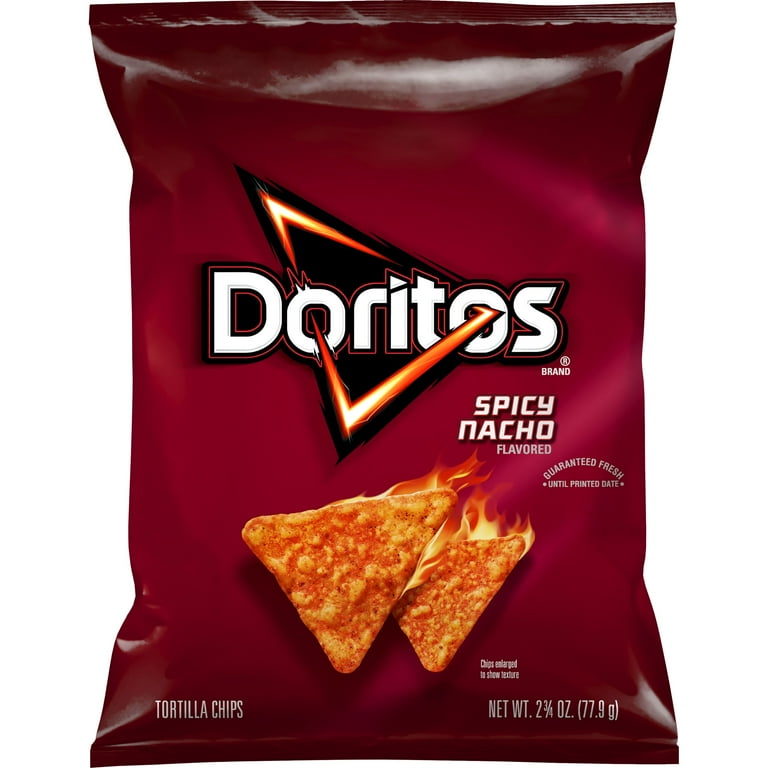The image is a detailed, photorealistic depiction of a small, single-serve bag of Doritos Spicy Nacho flavored chips, set against a stark white background. The bag's primary color is a maroon or burgundy that darkens slightly at the top and bottom. Adorning the front of the bag is the iconic Doritos logo with its distinctive triangle shape running through the O's. Beneath the logo, an image of two Doritos chips is prominently displayed, both emitting realistic flames that highlight the "Spicy Nacho" flavor. The chips themselves are orange triangles speckled with darker orange flecks. The text "Spicy Nacho Flavored," "Tortilla Chips," and "Guaranteed Fresh" are visible along with the net weight of 2 3⁄4 ounces (77.9 grams) in the bottom corner. The image of the bag appears almost photographic, though parts, especially near the top, seem slightly airbrushed, adding a touch of unreality to the otherwise vivid representation. Bits of glare can be seen on the bag, enhancing its realistic texture.